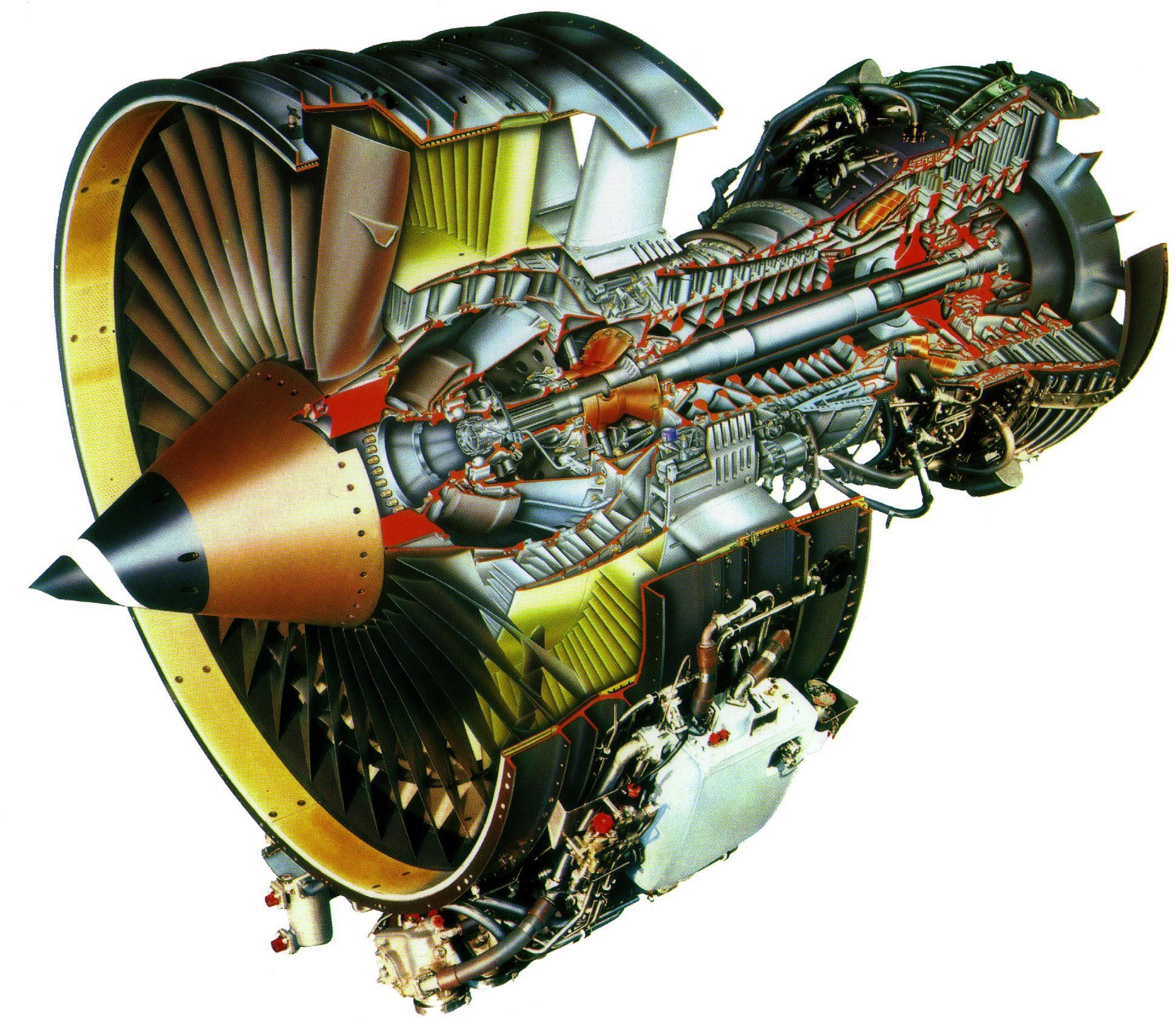A highly detailed, partially cross-sectioned diagram of a jet engine, revealing the intricate internal mechanisms. The front of the engine features a prominent cone with a black tip adorned with a white spiral, transitioning into a copper hue. Surrounding the cone are copper-colored fan blades. The interior showcases a complex array of components, including the compressor stages, combustion chamber, and exit vanes. Among the exposed elements are numerous metal tubes, shafts, valves, and yellow structures lining the fan's interior. The image, set against a blank background, uses color-coding to distinguish various parts, enhancing the visibility of the engine's sophisticated workings. This partial exposure allows for an educational glimpse into the otherwise concealed internal architecture of the jet engine.